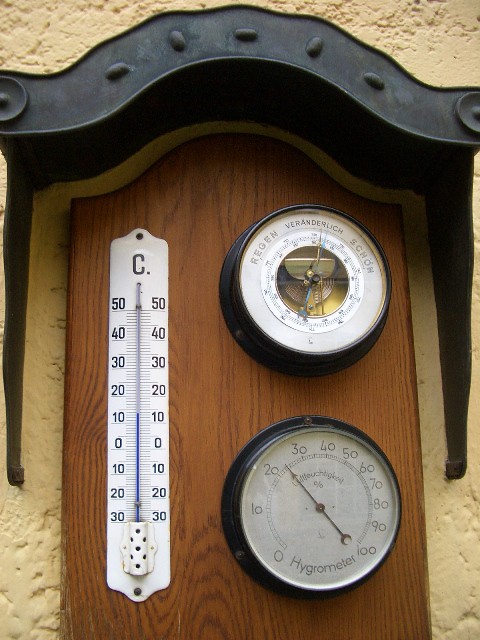This photograph depicts a weather station setup on a stucco exterior wall of a home. The station is mounted on a stained wooden board and features three distinct instruments, each with a specific function. The setup includes a thermometer with a hood-like black cover for protection against the elements. The thermometer displays a reading in Celsius, indicating a temperature of approximately 15 degrees. Below the thermometer, a round hygrometer measures the humidity, which is currently at 22%. Positioned above these instruments is another round meter featuring a copper center and the word "Redden" inscribed on it, although its specific purpose is not identified. Collectively, these instruments are installed to monitor and report various weather conditions.